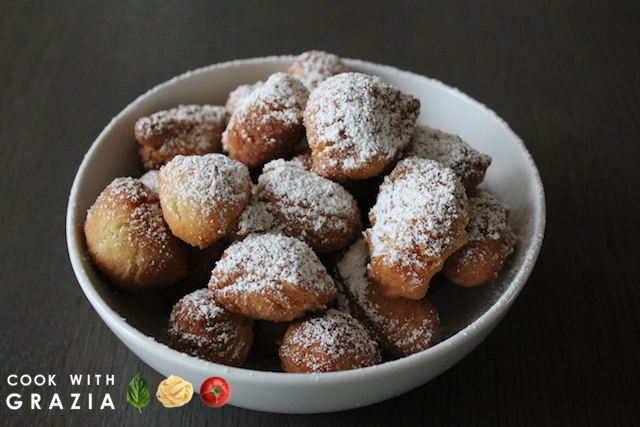The photograph features a white, circular glass bowl filled with small, round, tan-colored baked goods that resemble miniature donuts. Some of the items are oblong, adding visual variety. Each piece is generously dusted with powdered sugar, which also sprinkles the lip of the bowl, giving a fresh and inviting appearance. These sweet treats are set against a dark gray or charcoal-colored background, enhancing their golden hues. The setting is minimal and uncluttered, placing full emphasis on the delicious-looking baked goods. In the bottom left corner, "Cook with Grazia" is written in white letters, accompanied by three small icons: a green basil leaf, a rolled-up piece of pasta, and a tomato, suggesting a culinary context for the treats. This simple yet effective composition highlights the dessert and evokes a sense of freshly made, home-baked goodness.